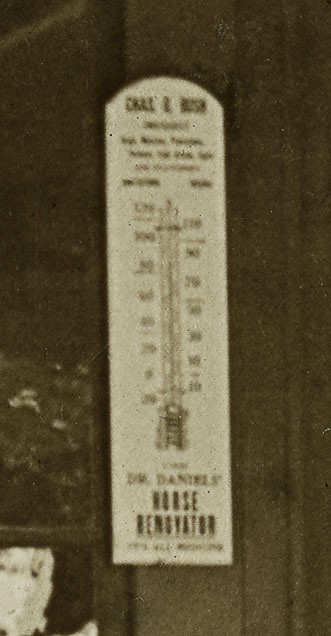The image features an old-fashioned thermometer mounted on a vertical wooden-paneled wall. The thermometer itself is white and contains mercury, visible as a shiny gray substance. It is calibrated in both Fahrenheit and Celsius. Although slightly blurred, a sign accompanies the thermometer, seemingly reading "Dr. Daniels Horse Benstator". The photograph is in grayscale, enhancing the vintage feel. In the far bottom left corner, there appears to be an object made of white material alongside a dark-colored box, with another rectangular object positioned above it.